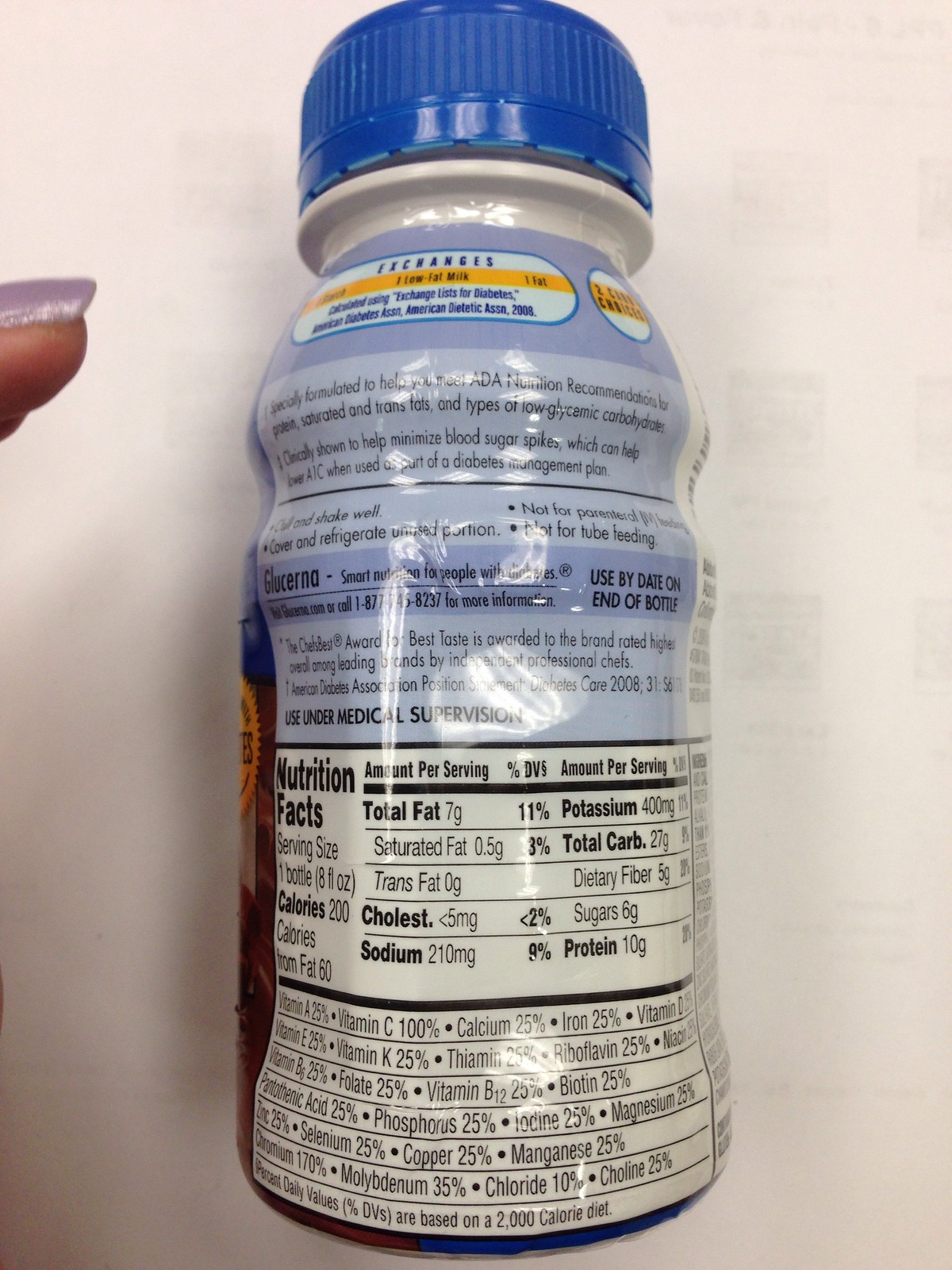The image depicts the back of a meal replacement or nutritional beverage bottle, likely a product named Glucerna, given the visible text "Glucerna, Smart Nutrition for People with Diabetes." The label details its nutritional content: each serving size is one bottle, which contains 8 fluid ounces. Nutritional values include 200 calories (with 60 calories from fat), 7 grams of fat, less than 5 milligrams of cholesterol, 400 milligrams of potassium, 27 grams of carbohydrates, 10 grams of protein, and 210 milligrams of sodium. The bottle is positioned lying down on a white surface. On the left side of the image, part of a woman's hand, with nails painted pink or purple, is partially visible.